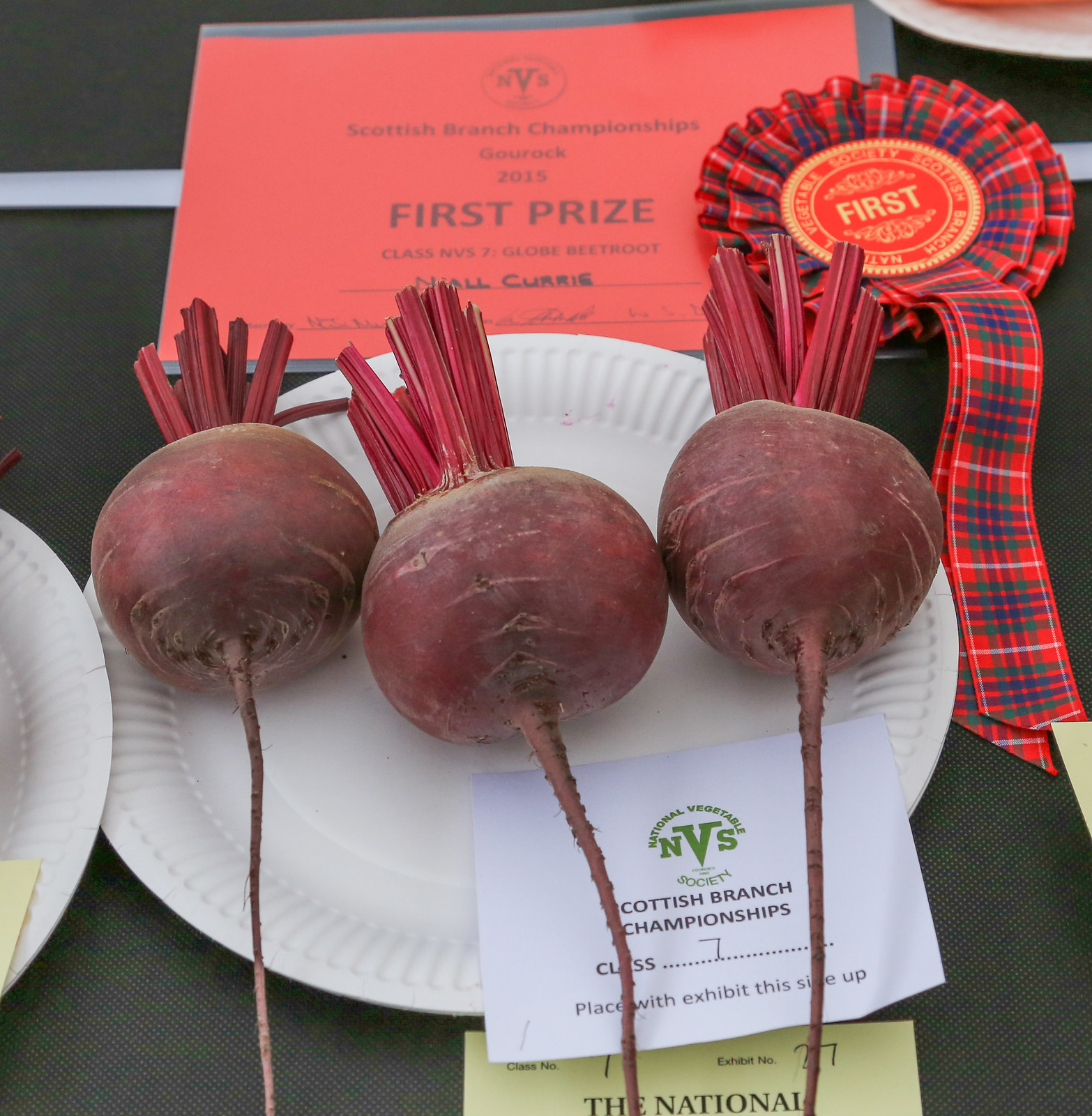In the image, a meticulously arranged white paper plate holds three large, dark purplish beetroots with vibrant pink stems, showcased for a judging competition. The background is a black table, enhancing the prominence of the prize-winning vegetables. Above the plate, a red laminated card prominently displays details in black font, reading "Scottish Branch Championships, Gourock 2015, First Prize, Class NVS-7, Globe Beetroot," with the winner's name, Niall Curry, inscribed below. Adjacent to the card, a red, green, and blue plaid first-place ribbon is prominently displayed, with "First" emblazoned in gold letters in the center. Additionally, a white card rests on the plate itself, reiterating the event's details with "Scottish Branch Championships, Class 7" visible. Partial glimpses of another paper plate and a yellow card with more text are visible to the left and beneath, respectively, hinting at further entries in the competition.